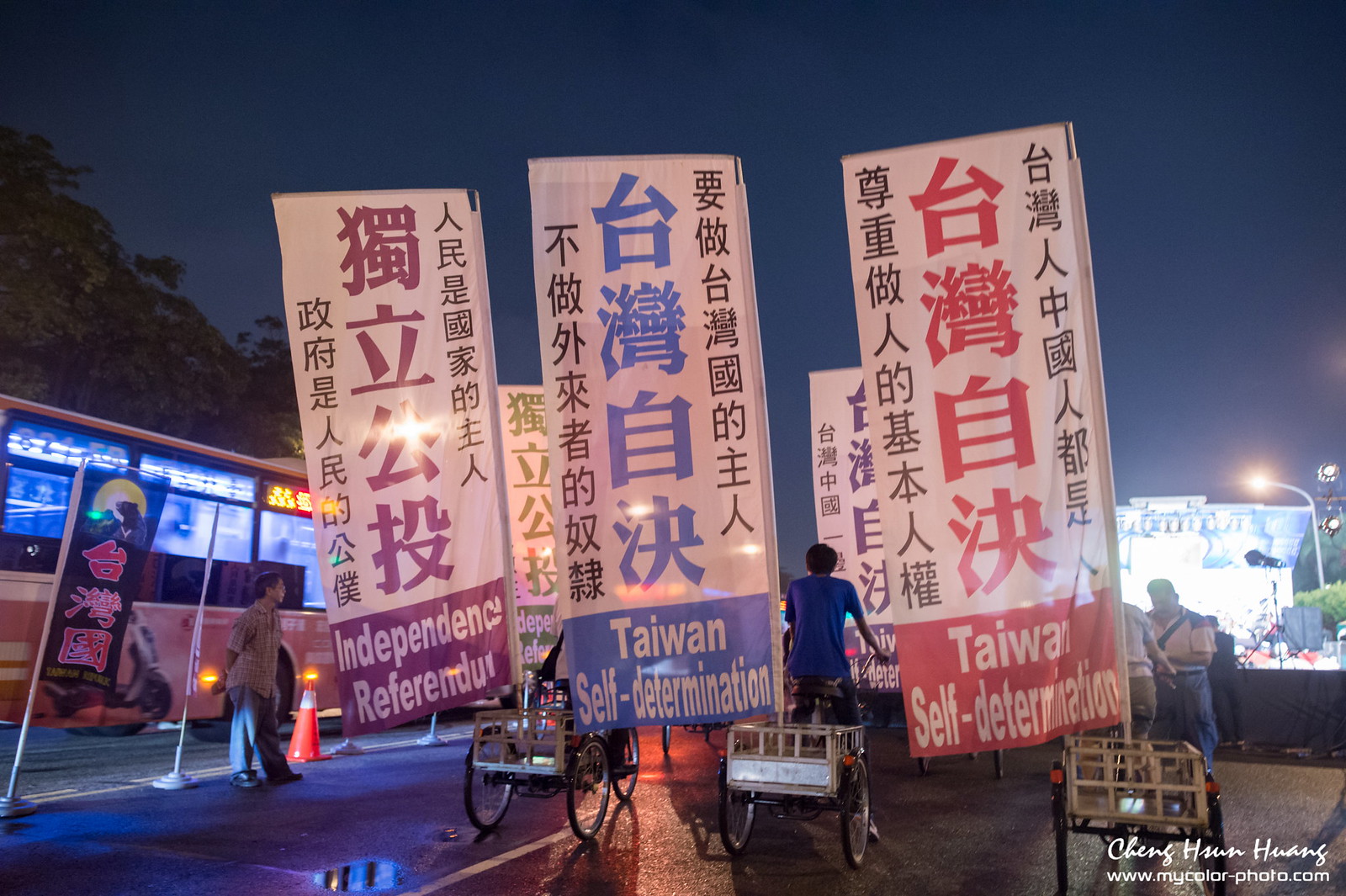This nighttime photograph, taken at an outdoor marketplace in Taiwan, beautifully captures a scene filled with vibrant activity and colorful displays. The main focus is on three people riding three-wheeled bicycles, each equipped with a tall flag. These flags, topped with traditional Chinese characters, also feature English text at the bottom. The left flag, on a purple background, reads "Independence Referendum," while the middle and right flags, on blue and red backgrounds respectively, read "Taiwan Self-determination." Additional flags are partially visible further ahead, but their details are obscured.

To the left of this procession, a partial view of a standard passenger bus, red and black in color, is apparent alongside a man with dark pants, shoes, and a plaid short-sleeved shirt. The backdrop features a stage, brightly lit, suggesting a lively event or parade. The street is adorned with various signs in colors like black, white, blue, pink, orange, and yellow, though some are blocked from view. Despite the crowd, it is predominantly men who are seen, though their features are not clearly visible. The bottom right-hand corner credits the photographer Cheng Huan Wang with the URL www.mycolor-photo.com. Surrounding the scene are street lights, lamp posts, a dark blue sky, and green leafy trees, adding depth and atmosphere to the lively Taiwanese streetscape.